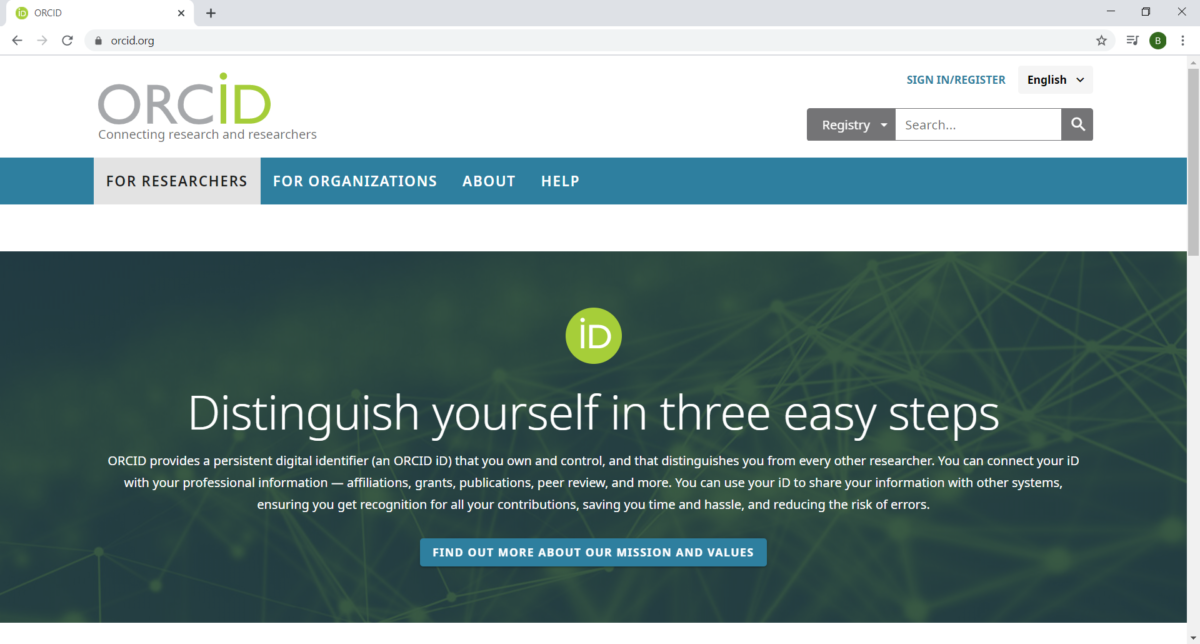The image depicts a detailed interface of the ORCID website, designed to connect researchers with research. At the top left corner, there is a white tab featuring a lime green circle with the letters 'iD' inside – 'i' in lowercase and 'D' in uppercase, both in white. This is followed by the bold, uppercase letters 'ORCID,' spaced out as O-R-C-I-D. 

Adjacent to this, a gray bar displays several control icons: a plus sign, a minus sign, two overlapping squares, and an 'X'. Below, there's a navigation line showing a dark gray left arrow and a lighter gray right arrow, along with a circular refresh icon, a lock symbol, and the text 'ORCID.org.' Continuing to the right, a star icon is visible, followed by several lines of type, and a blue circle featuring the letter 'B' above three vertically stacked dots.

Further to the right, the ORCID logo appears, with 'ORCID' split into 'O-R-C' in gray and 'iD' in lime green. Underneath, the tagline 'Connecting Research and Researchers' is prominently displayed. To its right, a blue 'Sign in / Register' option is present, accompanied by a gray dropdown box labeled 'English.' Adjacent to these elements, a gray box reading 'Registry' is positioned on the right side, near a white search box with an accompanying magnifying glass icon.

A blue banner stretches across the next line, starting with a slightly darker blue block. The words 'For Researchers' are inscribed in gray, followed by 'For Organization,' delineating different sections of the interface. Each element is meticulously arranged to facilitate easy navigation and access for researchers and organizations alike.